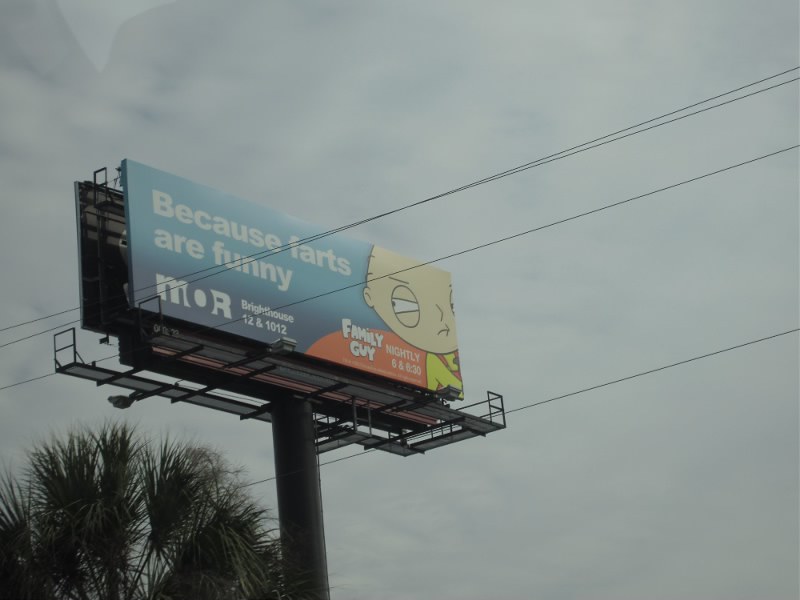This angled photograph captures a towering billboard set against a clear blue sky. In the bottom left corner of the image, a tall tree is visible, but the billboard itself surpasses the height of the tree. Power lines stretch diagonally across the frame, running from the lower left center towards the upper right, intersecting the image but not overshadowing the prominence of the billboard. 

The billboard features a bright blue background with an image of Stewie from Family Guy situated in the right corner. Dominating the left side of the billboard are the words "Because Farts Are Funny" displayed in large, bold white letters. In the lower left corner, it reads "MOR Brighthouse 12 and 1012." To the far right bottom, the text indicates the showtimes for Family Guy, stating "Family Guy Nightly 6 and 830." The overall scene combines elements of urban life with pop culture, all encapsulated in a bright and vivid composition.